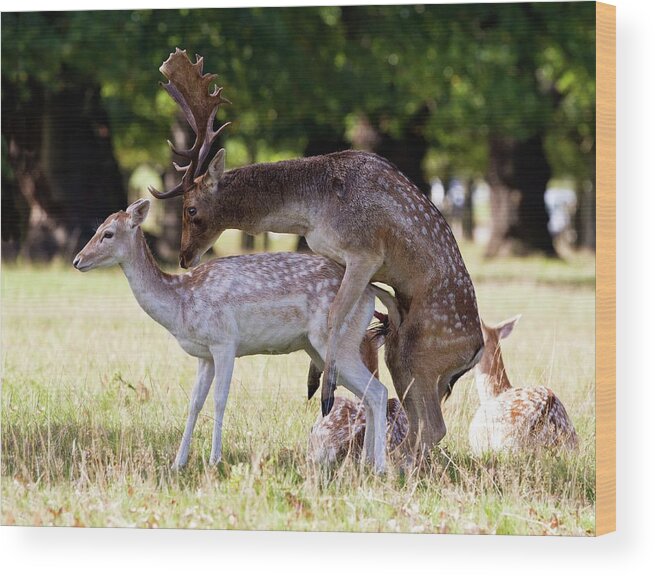In this wildlife photograph, taken in bright daylight, a male elk with large antlers and a dark brown coat speckled with white spots is attempting to mate with a smaller, lighter-colored female elk. The female, with a tan back, white spots, and a beige undercoat, lacks antlers and stands in front of the male who mounts her from behind, balancing on his hind legs. To the side, another female deer, also without antlers, lies on the green grass, looking away. The scene is set in a verdant grassy field bordered by a dense copse of green-leaved trees, all bathed in sunlight.